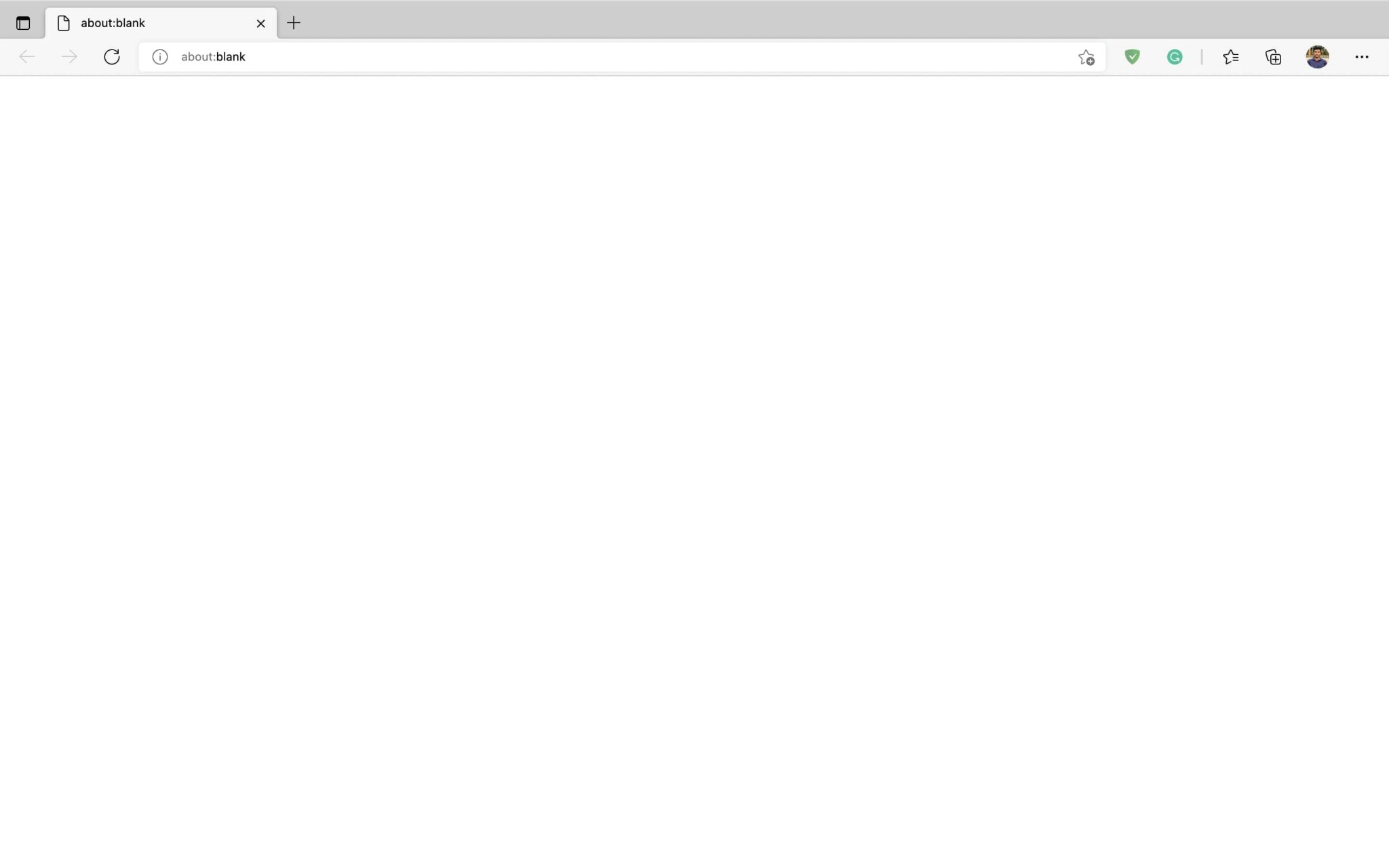Screenshot of a blank browser tab with a gray navigation bar at the top. The single browser tab on the left side is labeled "about:blank" and appears in a lighter shade of gray than the navigation bar. The URL bar also displays "about:blank." To the right of the URL bar are six icons: a star for bookmarks, a green shield, a teal circular refresh button, another star icon, a plus sign, a user profile picture icon, and a three-dot menu icon. The main content area of the browser is entirely white and blank.